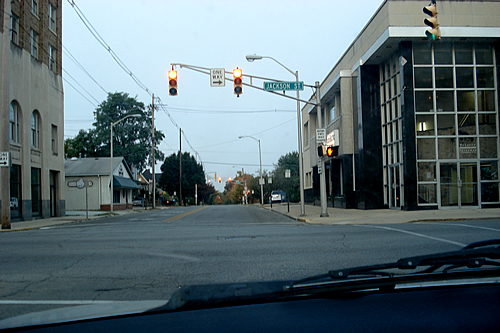A photograph is captured from the front windshield of a vehicle, evidenced by a small section of the dark gray or black dashboard and windshield wipers visible at the bottom edge of the frame. This image showcases a quiet intersection with a single car positioned at the traffic light. The traffic signal is red-rimmed but emits an unusual white light at its center. Positioned between the two traffic lights is a one-way sign directing to the right, next to a sign indicating "Jackson Street" against a green background. Off to the right side of the intersection stands a street light that is currently turned off. A green light can be seen shining through from the right-hand corner. The corner building appears to be a store, characterized by its first two floors consisting entirely of large, square windows and fully glass doors. As the street extends, the sidewalk runs parallel, lined by the building featuring black walls on the lower level and gray on the upper level.